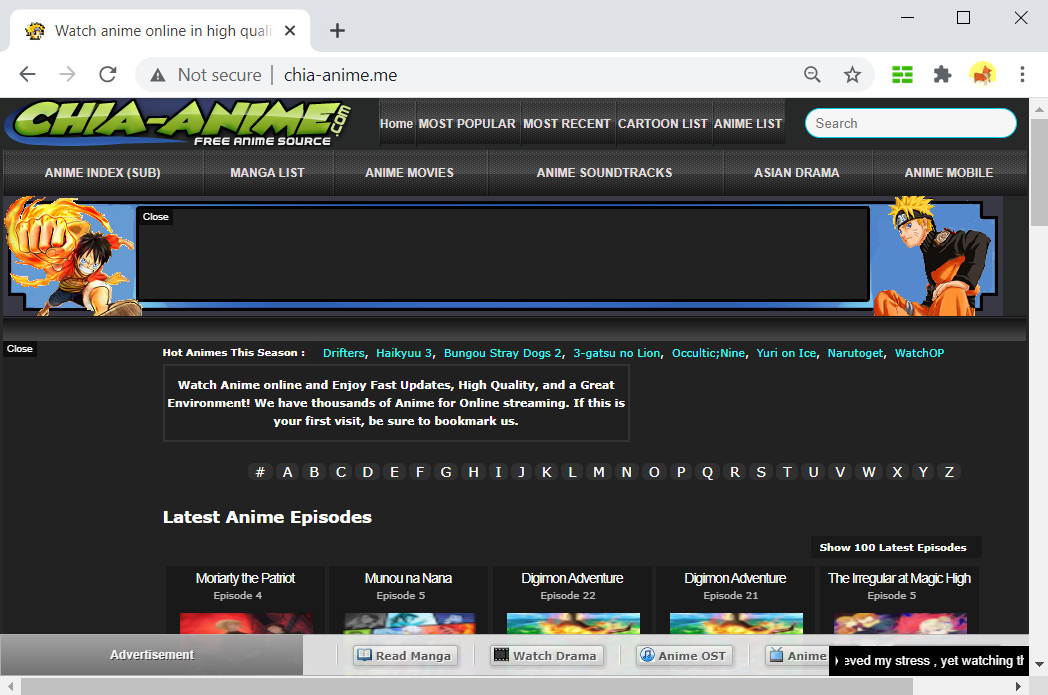Screenshot of an anime streaming website:

This panoramic screenshot captures a detailed view of an anime streaming website, hosted on a browser. At the very top, the usual browser controls (close, maximize, and minimize) are visible against a gray background. The browser tab is titled "Watch Anime Online in High Quality," but the text fades out towards the end. Next to the tab title, a black 'X' is present for closing the tab. The URL bar indicates that the website is "Not Secure" and is hosted at "chia-anime.me." Various browser icons are also visible, including a search magnifying glass, a star for favorites, forward and backward buttons, a refresh icon, a green bricks icon, a gray puzzle piece, a yellow semi-circle with something brown, and three vertically stacked gray dots.

The website itself prominently displays "Chia-Anime.com" in large, green, whimsical font at the top left, with "Free Anime Source" in white letters underneath, all against a greyish background. Adjacent to the main title is a blue swoosh design, enhancing the visual appeal.

Anime characters are featured on both sides towards the top of the page, nestled against a gray box, with a blue background behind them. Directly below the site title, a navigational alphabet from A-Z, including a pound sign (#), allows users to browse anime titles alphabetically. 

Centered on the page is a text box with white letters that reads: "Watch anime online and enjoy fast updates, high quality, and a great environment. We have thousands of anime for online streaming. If this is your first visit, be sure to bookmark us."

Further down, below the alphabet links, is a section labeled "Latest Anime Episodes" in white text. This area displays the names and episode numbers of various anime series, but only the top third of their corresponding pictures are visible.

At the very bottom left, there's a gray bar labeled "Advertisement" in white text. Adjacent to this, a white bar features multiple icons and links: "Read Manga" with a book icon, "Watch Drama" with a film reel icon, "Anime OST" with a blue icon, and "Anime" with a TV symbol. However, part of this area is obstructed by a moving black box with white text that reads "My stress yet watching," possibly a scrolling announcement or notification.

This detailed snapshot provides an intricate view of the anime website's layout and accessibility features, inviting users to easily navigate and explore a vast collection of anime content.